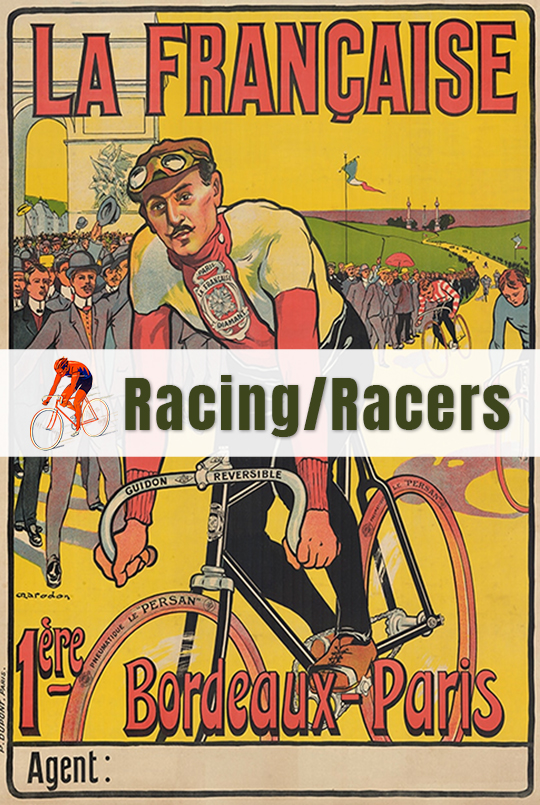The poster caption reads: 

"An eye-catching, retro-styled drawing depicts a cycling race poster with vibrant colors and a vintage feel. Dominating the top in large red letters is 'La Française'. Below it, a prominent cyclist is featured, riding a bike turned slightly left, adorned in a white shirt with long red sleeves, and a distinctive brown hat with goggles perched on the brim. He sports a small mustache and goatee. Around his neck hangs an emblem-laden accessory. A white band across the middle showcases text in black that reads 'Racing/Racers' alongside an image of another cyclist. The backdrop includes a yellow road lined with green grass and spectators, including notable landmarks such as the Arc de Triomphe on the upper left. Other cyclists trail behind the main figure. At the bottom of the poster, in red letters, it reads 'Bordeaux-Paris', with 'E-R-E' positioned to the left of the man’s bike tire and 'Agent:' marked in a small gray border on the left-hand side. The scene captures a vibrant and lively bicycle race, likely from the 1960s, brimming with a retro charm."